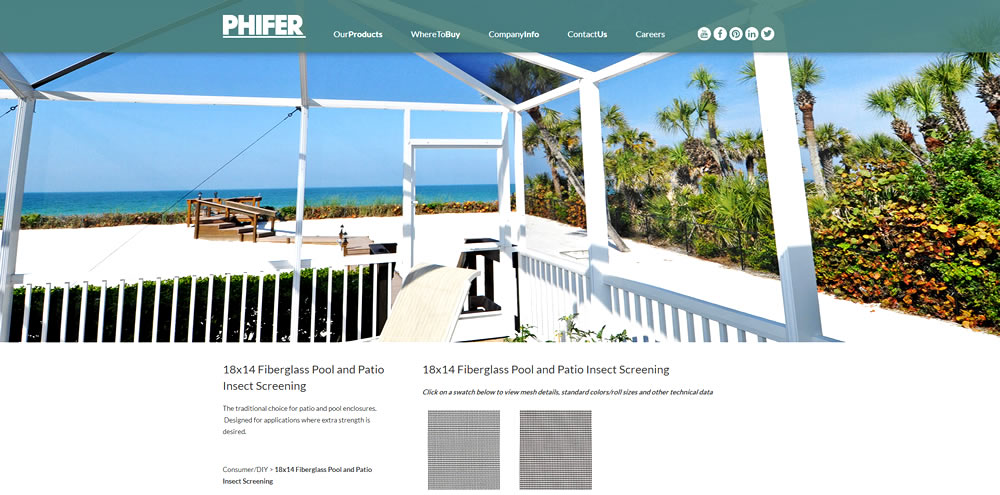Screenshot Ad for Pfeiffer Company

At the top of the page, the large text "Pfeiffer" is prominently displayed, underscored by a white line. Adjacent to the company name are navigation links in smaller text: "Our Products," "Where to Buy," "Company Info," "Contact Us," and "Careers," along with social media icons for Facebook, Twitter, Pinterest, and additional platforms.

Directly below this header is a sprawling photo of a deck area, which spans the width of the page. The deck features white flooring and white support beams, with a clear blue sky and a body of water visible in the background. The right side of the deck is bordered by lush tropical trees. Despite the focus on the deck, the product being advertised is "18 by 14 Fiberglass Pool and Patio Insect Screening," which is described as the traditional choice for patio and pool enclosures, designed for applications requiring extra strength.

Below the image, there are details about the insect screening, accompanied by the prompt, "Click on a swatch to view mesh detail, standard colors/roll sizes and other technical data." Two product choices are presented for the insect screening, although the mesh itself is not clearly visible in the photo, possibly due to the image's slight blur. The deck remains the central feature of the photograph.